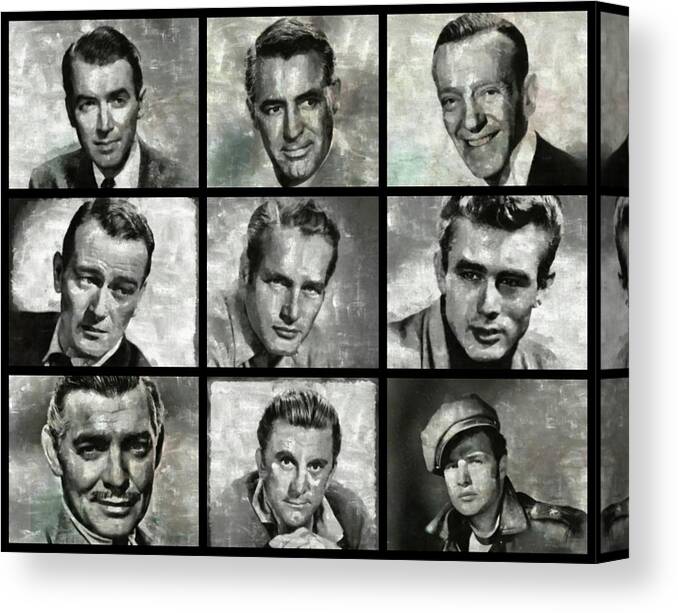The image is a stylized mosaic featuring nine iconic Hollywood actors from the classic era of the 1940s, 50s, and 60s. Each actor's black-and-white portrait has been given a watercolor painting effect, lending a unique artistic flair to the collection. Set against a green background, the portraits are neatly arranged in three rows, each with three actors. The top row features James Stewart, Cary Grant, and Fred Astaire. The middle row showcases John Wayne, Paul Newman, and James Dean. The bottom row includes Clark Gable, Kirk Douglas, and Marlon Brando. The mosaic is framed with black borders, creating a collector's edition aesthetic. Faces of additional actors can be glimpsed on the sides, hinting at a larger collection beyond the visible nine portraits.